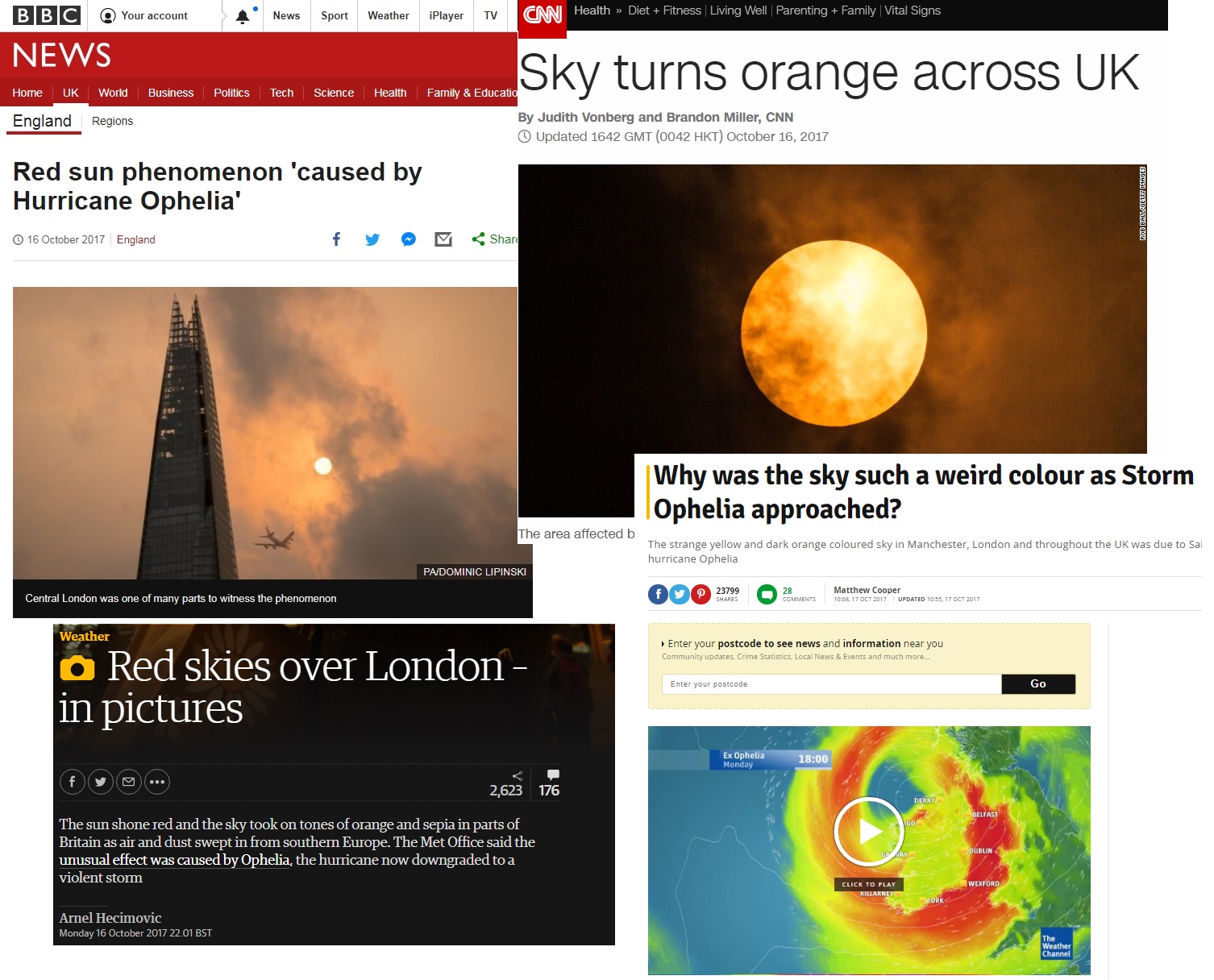Here's a detailed and cleaned-up caption for the described image:

---

The image depicts a webpage featuring various news and weather organizations reporting on the unusual red sky phenomenon caused by Hurricane Ophelia on October 16, 2017. 

1. **Top Left: BBC News** - The portion shows the sign-on page for BBC News with a red toolbar across the top, offering multiple clickable options. The highlighted headline reads "Red Sun Phenomena Caused by Hurricane Ophelia" with the date displayed as October 16, 2017. Under the headline, there is an image of a skyscraper, viewed from ground level looking upward. Next to the skyscraper, a large airplane is visible, along with the sun and several clouds.

2. **Top Right: CNN** - This section of the webpage is displaying the CNN news site. The headline states "Sky Turns Orange Across the UK," accompanied by an image of a sun partially obscured by clouds. The subheadline reads "Why Was the Sky Such a Weird Color as Storm Ophelia Approached?"

3. **Bottom Left: Weather Website** - Below the BBC News section, there is a weather website featuring the headline "Red Skies Over London in Pictures," followed by descriptive text on the occurrence.

4. **Bottom Right: Weather App** - The last portion appears to be a weather app interface, allowing users to enter their postal code to receive weather updates. The interface features a multicolored weather map.

---

This detailed caption encapsulates the essence of the visual information displayed on the webpage, providing a clear and descriptive overview.